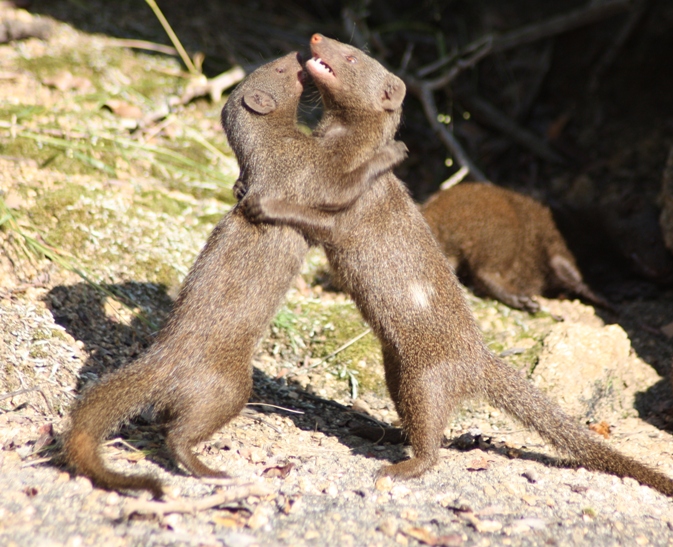The image captures a dynamic scene featuring three small, brown furry mammals, possibly weasels or mongooses, set against a mixed background of grass, dirt, and scattered rocks. The two animals in the foreground are standing on their hind legs, with their front legs wrapped around each other in a posture suggestive of wrestling or playing. They have long tails, red noses, and tiny red eyes, with visible white fur around their ears. One of the foreground animals is baring its teeth, adding a sense of action to the scene. Shadows cast by the animals and the sun interplay on the ground. Positioned slightly behind them, a third animal, facing away and identifiable only by its dark brown fur and black feet, adds depth to the composition. In the background, the left side shows a darker area that might be the base of trees or shrubs, with an indistinct section of shadow and sticks occupying the upper right corner, hinting at a forested environment.